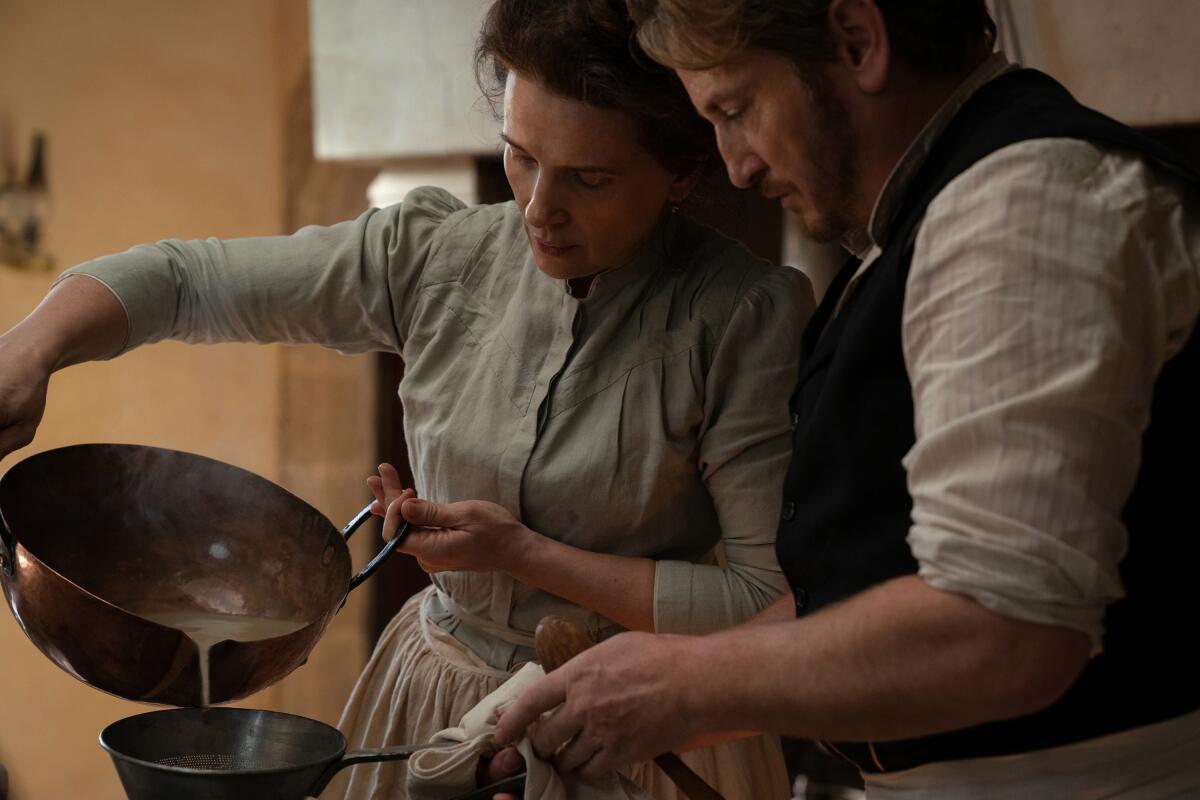In this detailed image, a middle-aged man and woman are pictured together, seemingly engaged in a cooking task. The woman, positioned on the left, is dressed in an older-fashioned outfit comprising a light green or possibly light blue-gray button-up blouse with three-quarter sleeves that end past her elbows, and a tan skirt tied around her waist. Her dark hair is styled in a way that might resemble a pilgrim’s hairdo. Beside her, the man, on the right, has brown hair and a beard. He is wearing a white, striped long-sleeve shirt with the sleeves rolled up to reveal his hairy forearms, along with a black vest.

The woman holds a large metal bowl with handles, from which she is pouring a dark cream-colored liquid into a smaller metal pot. The male counterpart holds this pot with a white towel, indicating it might be hot. The pots present a bronze or cast iron appearance. This scene seems to be set in a kitchen, hinted at by the beige-colored walls in the background, possibly suggesting an indoor environment. Both individuals appear to be in a serious yet focused collaboration, engrossed in their culinary activity.